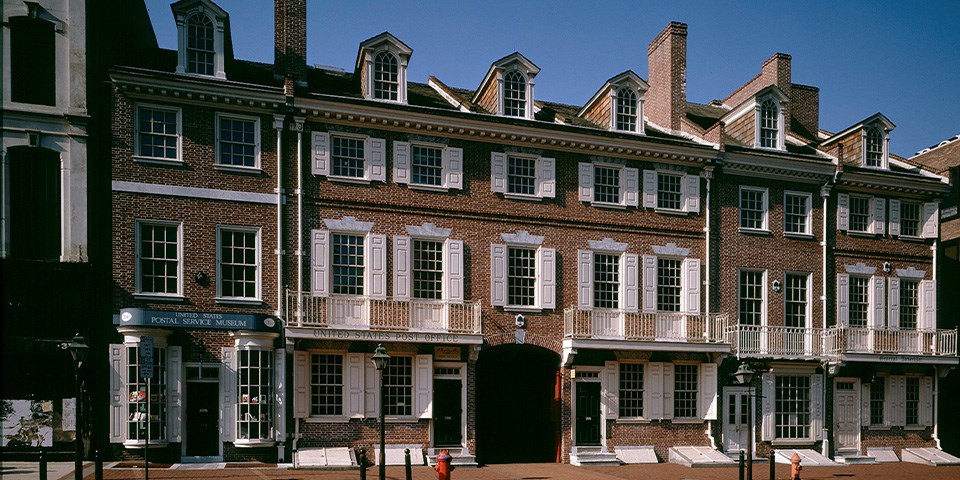The image is a photorealistic digital photograph of a city street showcasing a large, four-story building, though only three stories are accessible. The building, crafted from brown bricks, extends from the right to the left-hand side of the image in a continuous row of connected structures. Each floor contains white windows adorned with matching white shutters. The street level offers a variety of entrances and archways, including a prominent shop on the left bearing a sign reading "Postal Service Museum" in white letters on a blue background. The main entrance features a distinctive archway with red inner walls. The scene is bathed in the bright blue of the sky above, accentuating the brown roofs and the two chimneys seen towards the right side of the image. The ground is paved with brown stones, adding to the historic architectural feel, and the street is lined with black streetlights. A fire hydrant and a few additional street signs also make an appearance in this rich, varied scene colored in brown, white, blue, red, and hints of orange.